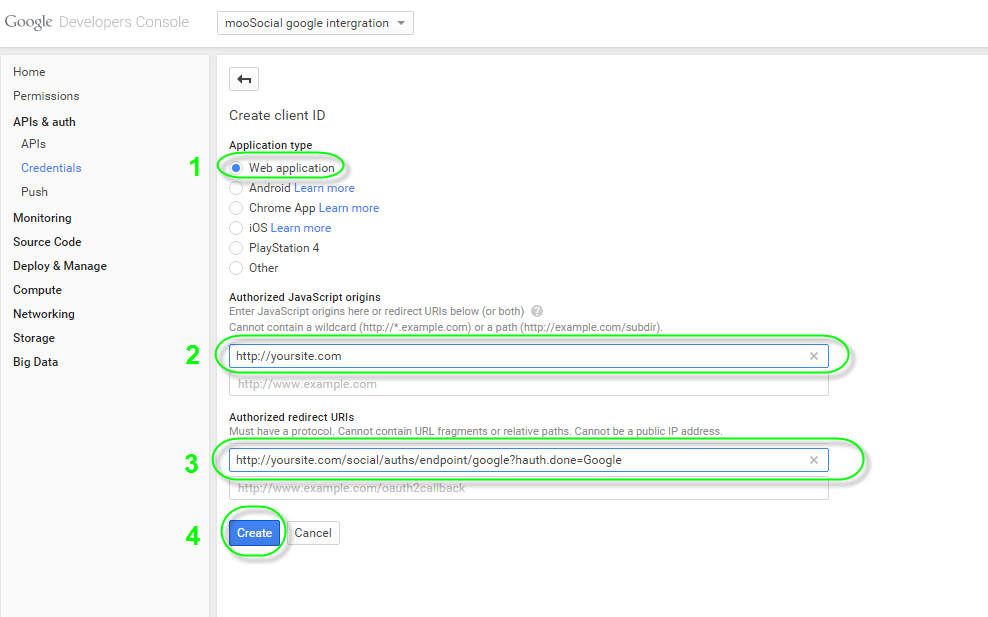This screenshot depicts a segment of the Google Developers Console interface, presented against a clean white background. In the upper left corner, "Google Developers Console" is prominently displayed. Adjacent to it on the right is a dropdown button labeled "Moo Social Google Integration."

On the left side of the screen, a vertical navigation menu is shown, featuring the following options: Home, Permissions, APIs and Auth, APIs, Credentials (highlighted in blue), Push, Monitoring, Source Code, Deploy and Manage, Compute, Networking, and Storage and Big Data.

To the right of the navigation menu, there is a section dedicated to creating a Client ID. It includes the following steps: 
1. Application type
2. Authorized JavaScript origins
3. Authorized redirect URIs

Beneath these instructions, a prominent blue "Create" button is encircled by a green outline, inviting users to complete the setup process.